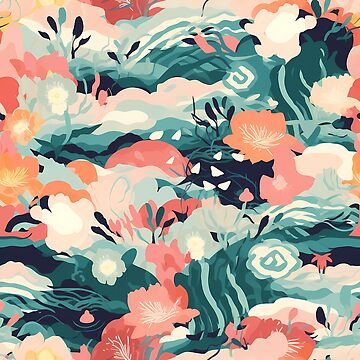This abstract painting captures a highly stylized waterscape adorned with various flowers and foliage. The water ranges from light to dark blue with shades of green, creating a dynamic and unpredictable scene, accentuated by the appearance of wind-blown petals. The flowers, which are scattered from the top to the bottom of the composition and include reeds on the top left, come predominantly in hues of orange, pink, and coral with lighter centers. Despite their generic shapes, the flowers and foliage are identifiable through their vibrant colors and flat forms, lacking broad leaves. Some flowers appear on the bank to the left, while others seem to be disintegrating, their fragments buoying upon the water surface. The color palette includes black, blue, green, pink, orange, coral, white, and off-white, contributing to the painting's intricate and old-fashioned aesthetic.